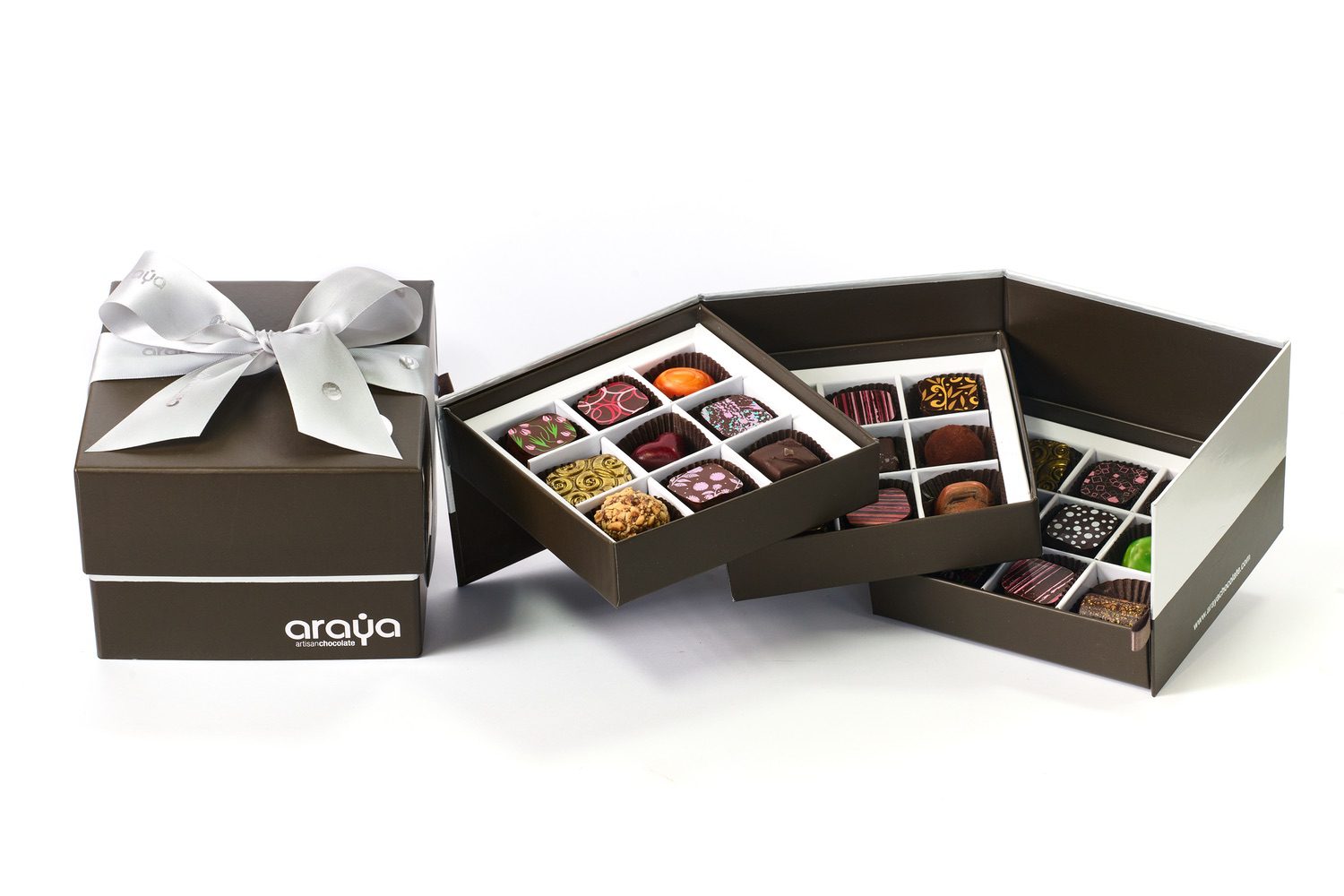This image showcases an elegant display of specialty chocolates from Araya. On the left side, there is a sealed, brown lidded box adorned with a hand-tied white bow and the Araya logo in white font at the bottom right corner. The right side reveals the contents of an opened, tiered box of chocolates. This box, which unfolds from the side, has its top lid removed to expose three staggered, brown trays with white trim. Each tray contains nine intricate truffle and brownie bites, arranged in a tic-tac-toe grid. The chocolates vary in shape, with some square and some round, featuring an array of vibrant colors and detailed patterns, including floral designs, stripes, and abstract art. Nestled in plastic accordion paper cups, some of the chocolates are adorned with nuts or painted surfaces. The arrangement creates a cascading effect, with the top tray leaning to the left, the middle tray slanted and exposed, and the bottom tray still within the box. The predominant colors in the image are chocolate brown and white, highlighted with accents of pink, green, orange, and yellow.